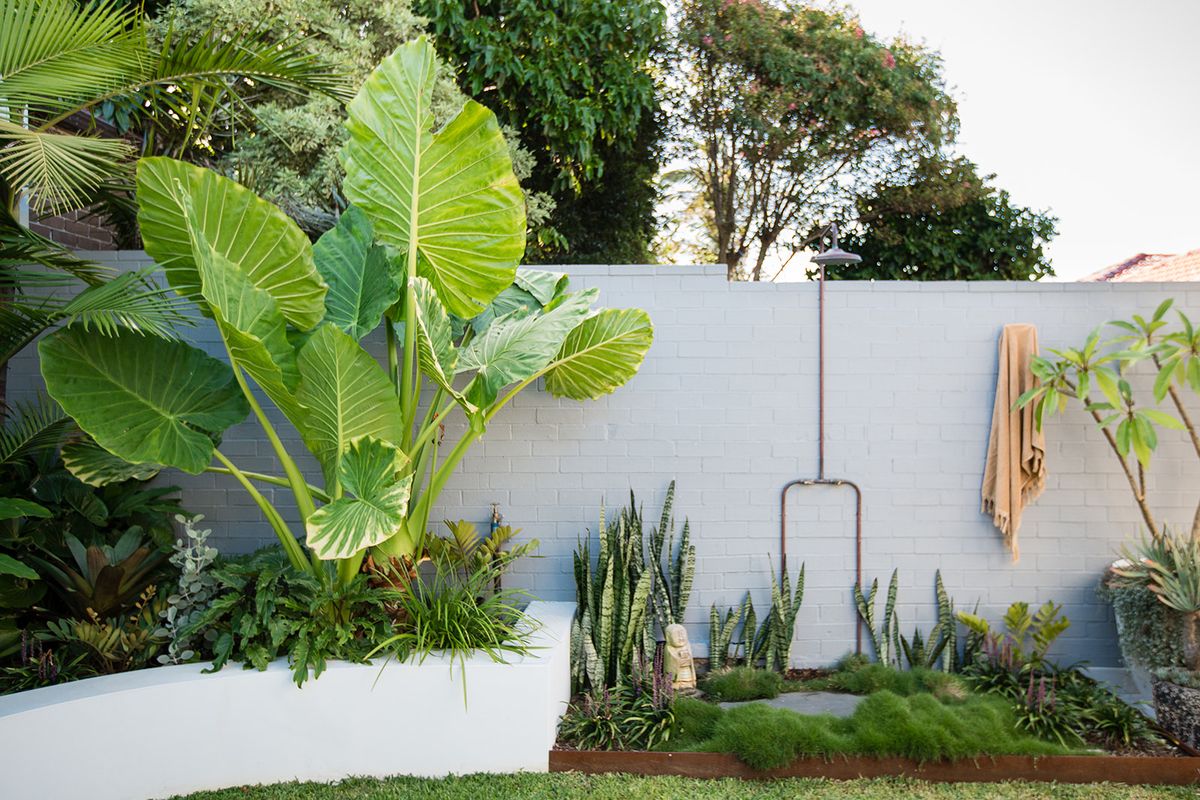The image is a detailed photograph of a well-manicured backyard garden or flower bed, framed as a horizontal rectangle. Dominating the center of the scene is a white or possibly gray brick retaining wall that spans across the entire background, separating different sections of the yard. To the left side of the image, there's a shorter border enclosing a flower bed filled with enormous elephant ear plants, their gigantic fronds making a striking visual impact. Above them, a palm leaf protrudes from the top left corner, adding to the lush tropical vibe.

In the bottom part of the image, a white garden statue with a carved human figure stands out, positioned near a small patch of moss and an approximately 8-inch high red brick wall on its right. The foreground also includes a very tightly cropped, short lawn area. The backdrop above the retaining wall reveals treetops, adding height and depth to the scene.

Additional details include a towel hanging on the wall near the right center of the image, adjacent to an outdoor shower head and its accompanying pipes to the left of the towel. The photograph, taken outdoors in daylight, showcases a vivid palette of green, dark green, white, gray, orange, brownish red, and brown, highlighting the vibrant and meticulously arranged landscaping of this backyard space.